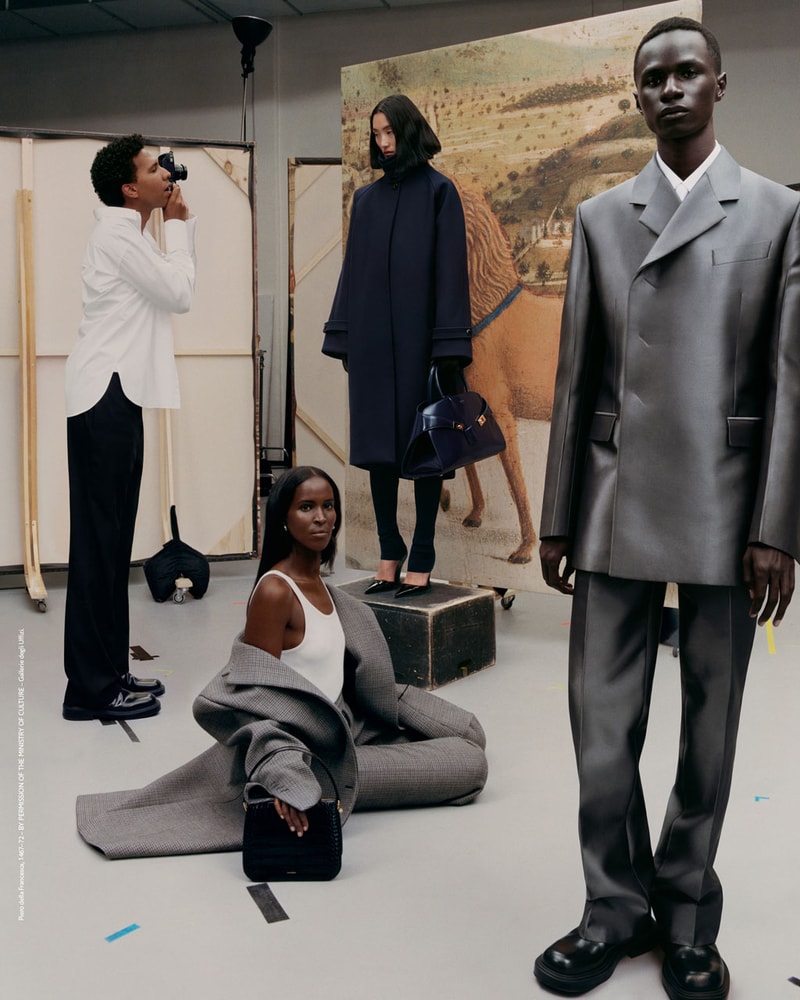In this detailed photo, a professional fashion shoot is underway. At the center, a photographer, donned in a crisp white long-sleeve collared button-down shirt, black slacks, and black shoes, holds a camera up to his eye, capturing the model in front of him. The model, an Asian woman with long black hair, is striking a pose while standing on a black wooden trunk. She is dressed in a navy blue coat, black pants, and black heels, holding a navy blue leather handbag. Behind her, a large painting depicting a lion and a green countryside serves as the backdrop. 

On the floor to the left, a stunning black model with long black hair sits elegantly. She is attired in a sophisticated gray coat and gray pants, complemented by a white sleeveless tee and holding a black purse. 

To the right, another man in a metallic-like gray suit with black shoes and thin black hair stands, watching the scene intently. This fashion shoot meticulously showcases the outfits and accessories, blending the models' poise with the creative backdrop.